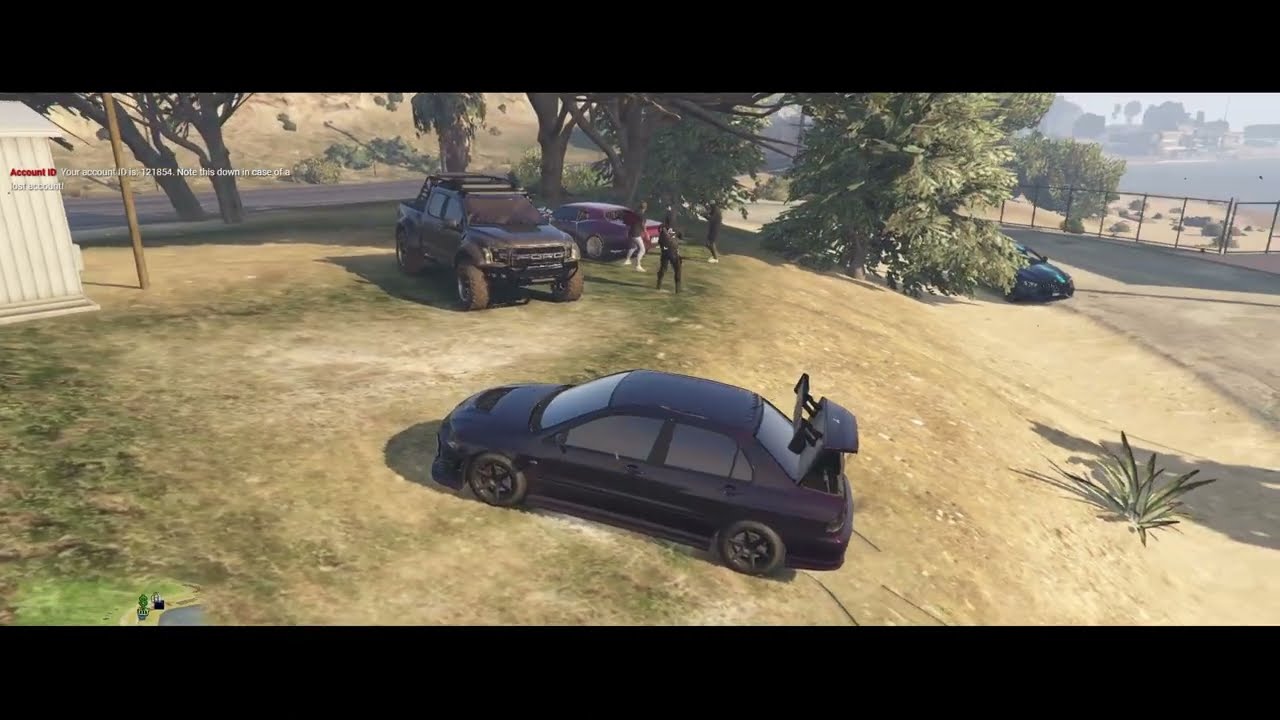The image is a highly detailed screenshot from the video game Grand Theft Auto (GTA). The scene is set outdoors, in the middle of the day, featuring a grassy and slightly hilly terrain with patches of dirt and yellow grass. In the foreground, there is a black Mitsubishi Lancer Evolution 9, commonly referred to as the Evo 9, with its trunk open and a prominent airfoil mounted on it. The car casts a noticeable shadow on the ground.

Adjacent to this car, partially hidden by trees with dark green leaves, is a 4x4 Ford parked under the trees, followed by a vintage car behind it with silver wheels, suggesting an eclectic mix of vehicles. Further in the image, a truck is emerging from behind the trees with a distinctive rail attached to its bed. There are also several people standing near the vehicles, dressed in dark-colored outfits, adding a sense of activity to the scene.

To the right, there is a paved road that curves around the hill where the cars and people are situated. Beyond this road, there is a fenced area with a light pole nearby. In the distance, the scene includes a hazy view of a farm, a metal shed, and a meadow, emphasizing the rural setting. A body of water is visible in the top right corner of the image, bordered by shrubbery and sandy areas. The entire image is framed with a black border at the top and bottom, reinforcing the screenshot's video game origins.